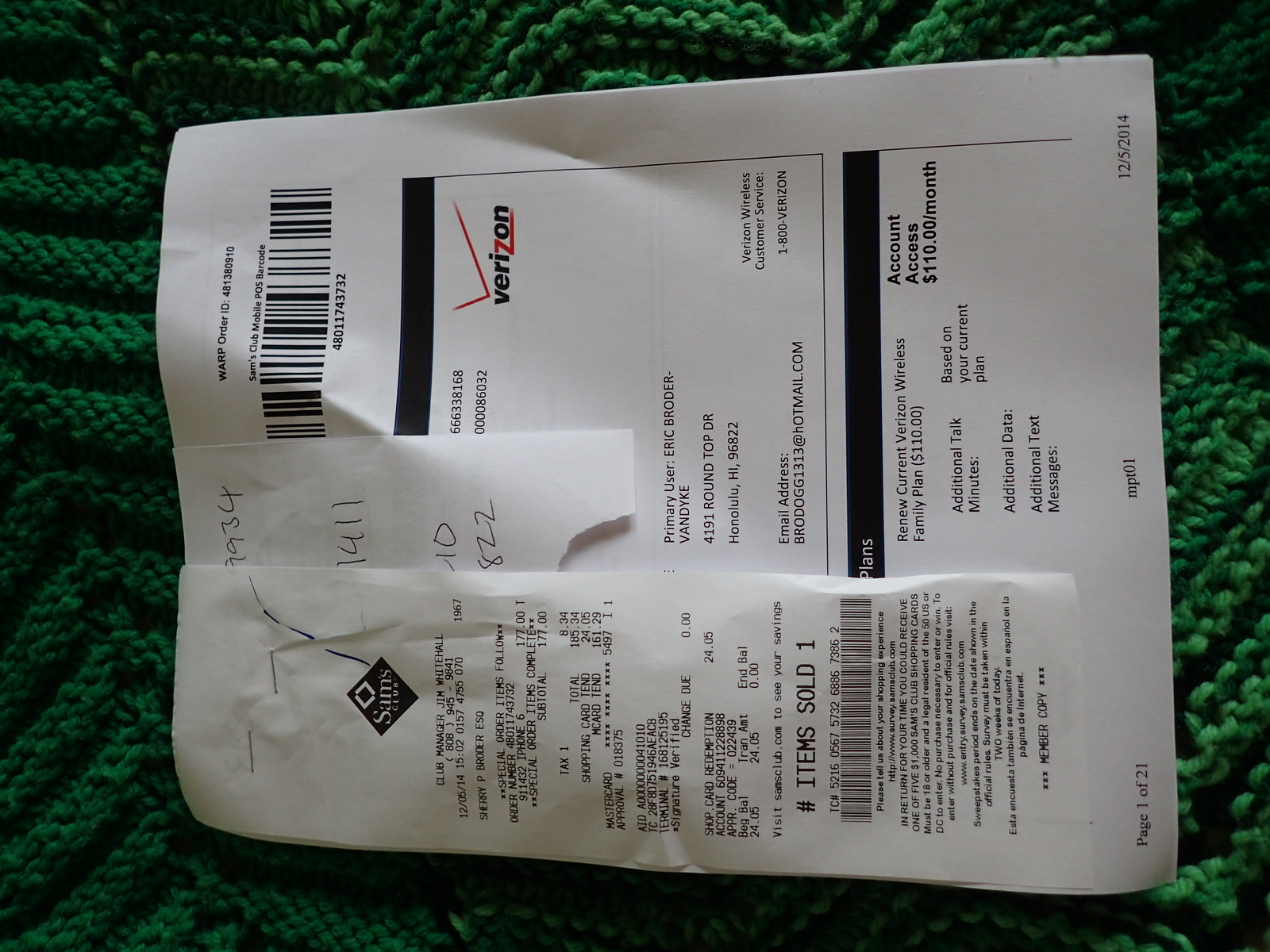In the image, a receipt from Sam's Club is prominently displayed on the bottom left, clearly marked with "item sold number one." This receipt is stapled to a larger, white Verizon document, which features intricate details such as account numbers, a customer’s email, address, and phone bill information. The Verizon logo is mostly in black, except for the letter 'Z,' which is highlighted in red with a check mark over it. Additionally, another small piece of paper with handwritten numbers is tucked between the Sam's Club receipt and the Verizon paper. The entire assemblage lies on a green, chunky knitted afghan, and the image appears to have been taken sideways, rotated 90 degrees counterclockwise, adding a unique perspective to the composition.